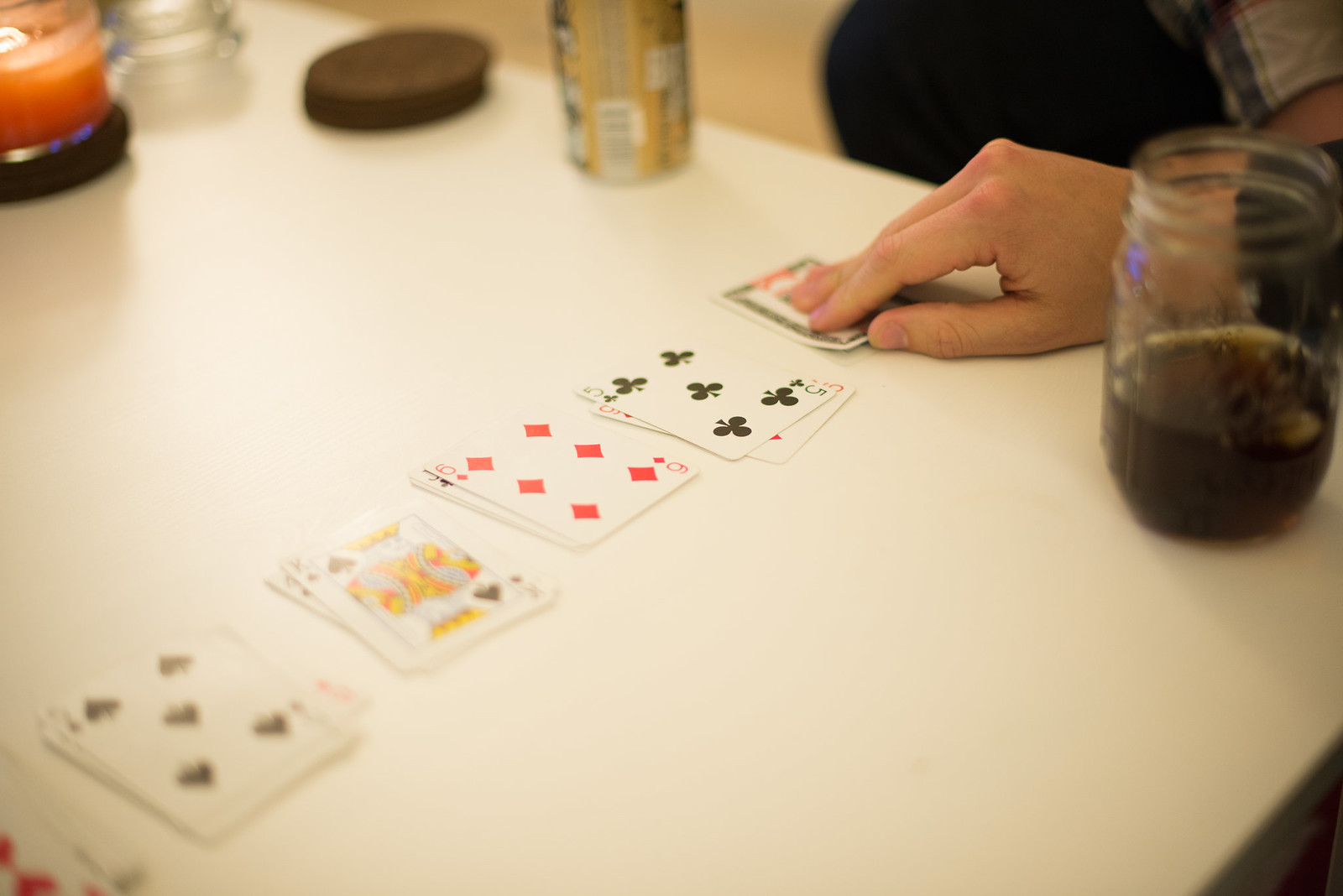In this captivating photograph, we see a close-up view of a card game in progress on a pristine white tabletop. Stacks of cards are meticulously laid out in a horizontal row across the table. In the foreground, a clear mason jar containing a cola drink adds a refreshing touch to the scene. Just behind the jar, a man's hand, clad in a dark long-sleeve shirt, is poised over one of the cards, with his thumb under the border and fingers atop, suggesting he's about to turn it over.

The table also features an aluminum can, slightly blurred, perhaps indicating a beer or soft drink. Beside the can is a stack of dark brown, round coasters neatly arranged. Dominating the center of the table is an orange candle housed within an elegant black candle holder, casting a warm ambiance over the setup.

The row of cards begins with a five of spades, followed by a king of spades, a six of diamonds, and a five of clubs. The identity of the card that the man is about to pick up remains a mystery, adding an element of suspense to this detailed and engaging scene.